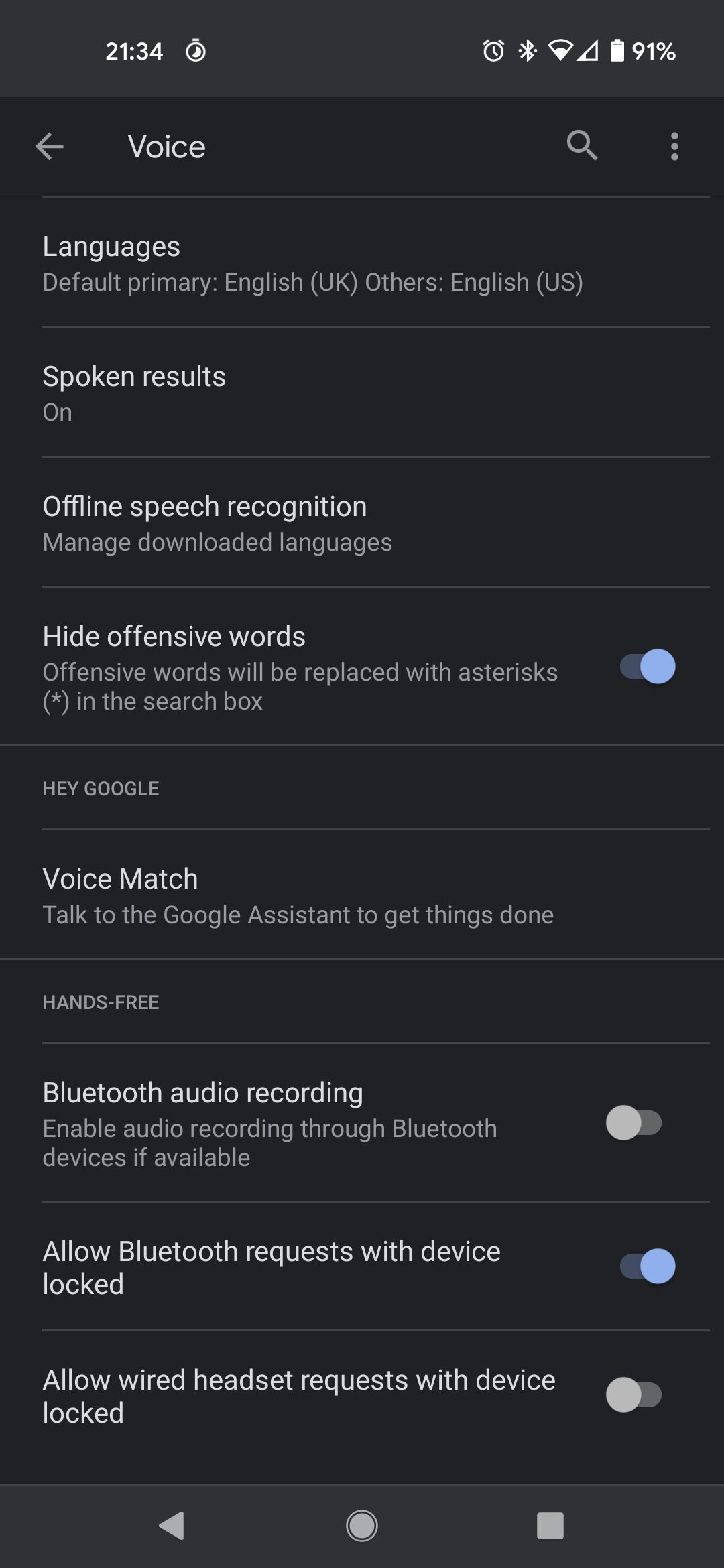**Caption: Detailed Screenshot of Phone Voice Settings**

The screenshot presents the voice settings menu of a phone, characterized by a very dark gray, almost black background. At the very top, a slightly lighter dark gray banner frames various status icons.

**Top Status Bar:**
- **Time:** Displayed on the top left, the time reads 21:34.
- **Icons from Left to Right:**
  - A quarter-filled clock icon, possibly indicating a timer.
  - An alarm clock icon, suggesting an active alarm.
  - The Bluetooth icon.
  - The Wi-Fi icon.
  - The carrier signal icon, indicating a signal strength of about 10 to 20%.
  - A battery icon displaying 90% charge.
  - The text "91%," confirming the battery status.

**Main Settings:**
- **Navigation and Header:**
  - A gray back arrow on the left.
  - The title "Voice" centrally positioned.
  - A search magnifying glass icon.
  - Three vertical dots indicating a menu.

Under the header, the settings are listed in white text with gray selections:

1. **Languages:**
   - Default Primary: English (UK).
   - Others: English (US).
   
2. **Spoken Results:** On.

3. **Offline Speech Recognition:**
   - Manage downloaded languages.

4. **Hide Offensive Words:**
   - Offensive words will be replaced with asterisks (*).
   - Toggle: On (blue).

5. **Hey Google:**
   - Voice Match: Talk to Google Assistant to get things done.

6. **Hands-Free:**
   - Bluetooth audio recording:
     - Enable audio recording if your Bluetooth device is available.
     - Toggle: Off (gray).
   - Allow Bluetooth request with device locked:
     - Toggle: On (blue).
   - Allow wired headsets with device locked:
     - Toggle: Off (gray).

**Bottom Controls:**
- A gray triangle pointing left.
- A circle within another circle resembling a record button.
- A gray square representing a stop button.